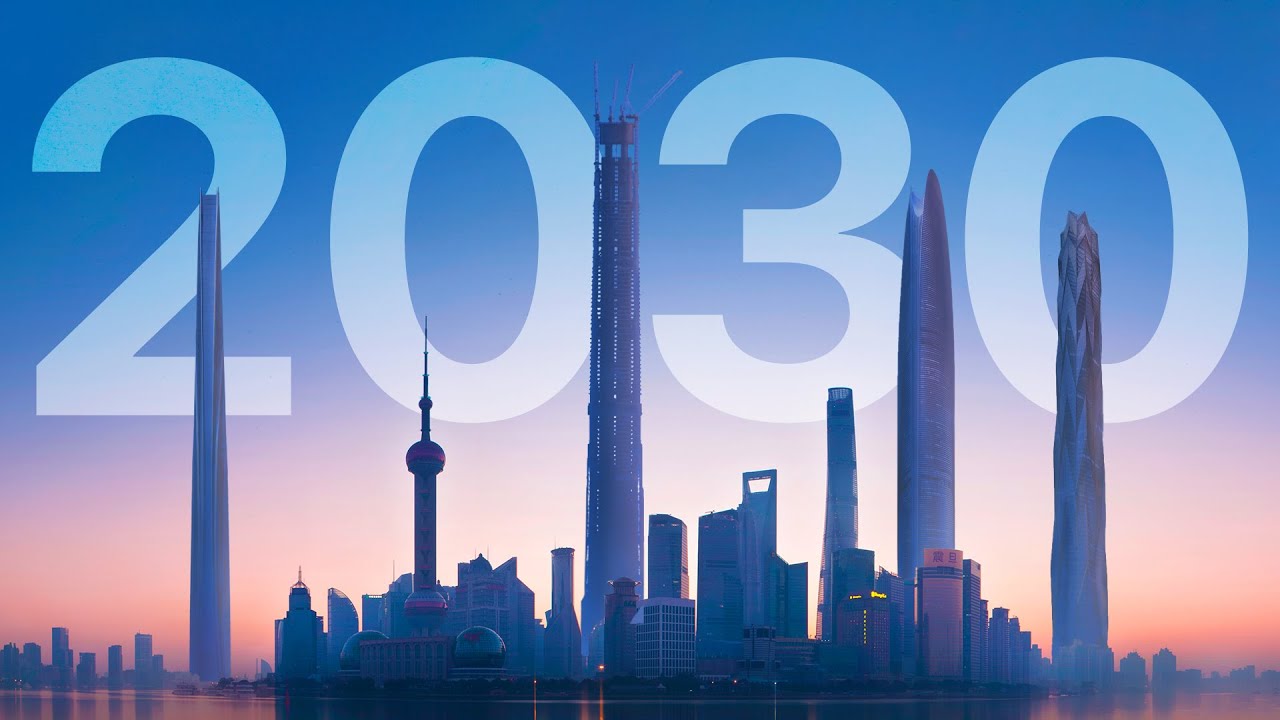This wide rectangular image is a stunning artist's depiction of a futuristic skyline set in the year 2030, prominently displayed in large numbers spanning the background. The scene is dominated by numerous sleek, symmetrical skyscrapers, with a few towering structures standing out, including one cylindrical building capped with a needle-like spire. Smaller buildings cluster at the base, completing the ultramodern cityscape. The skyline is set against a serene body of water, likely a bay, with the perspective taken from the water's edge. The lighting suggests dusk, casting a gentle, warm glow of pinks and oranges from the setting sun, which contrasts beautifully with the predominantly pale blue sky. Delicate hints of smog add a touch of realism to this visually striking and imaginative portrayal of urban architecture in the future.